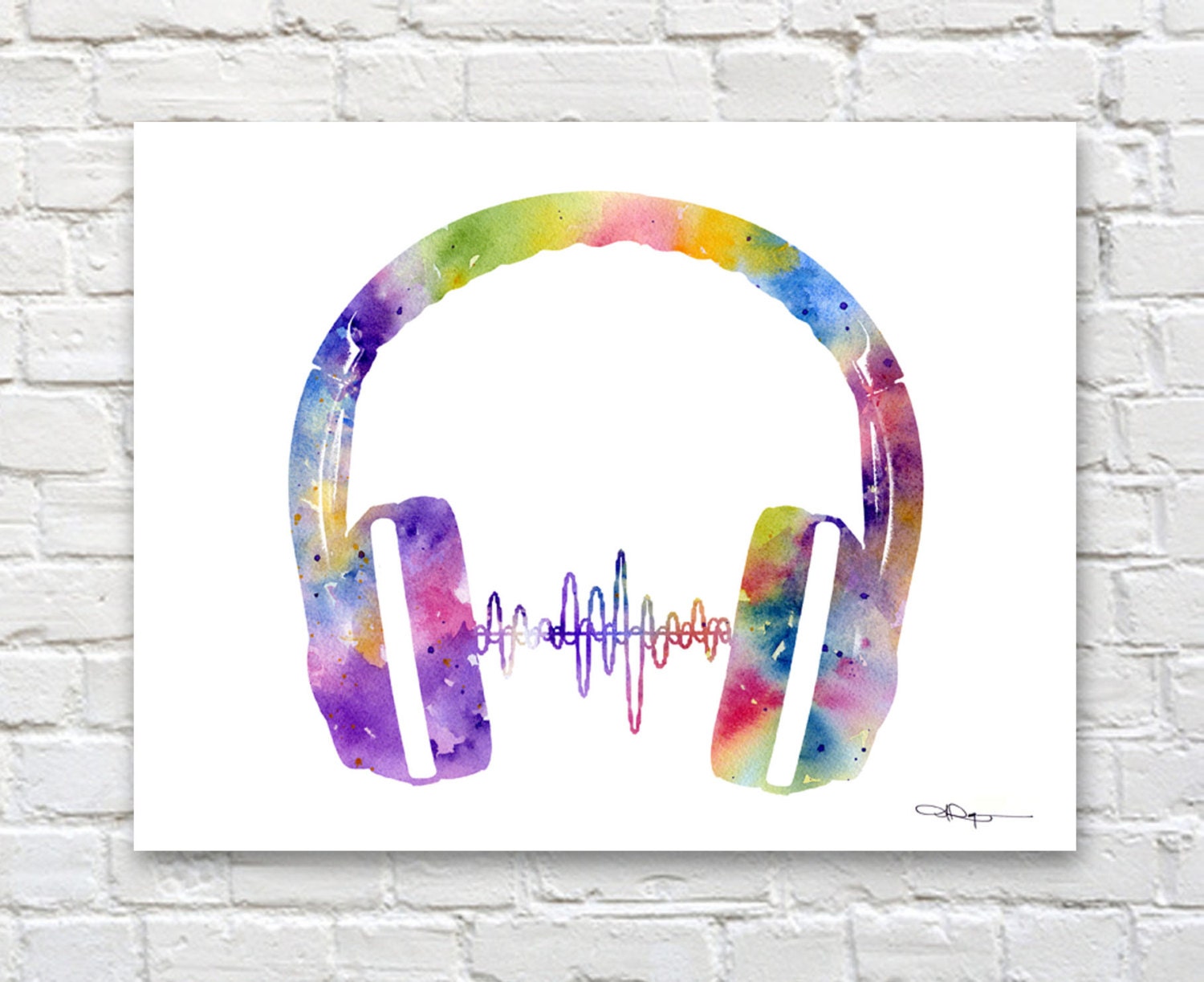Displayed against a white painted brick wall is a striking piece of art on a white rectangular canvas, oriented horizontally. The artwork features a vivid watercolor depiction of a pair of headphones, characterized by their intricate rainbow color scheme. The headband showcases a blend of hues ranging from yellow, blue, and purple to green, peach, orange, and yellow, culminating in a vibrant, psychedelic pattern. The earpieces themselves are also filled with a similar array of colors, creating a visually captivating effect. Bridging the two earphones is a series of multicolored sound waves, artistically rendered in shades transitioning from purple to red, green, and yellow, symbolizing the transmission of sound. Adding a final touch of authenticity, a signature adorns the bottom right corner of the canvas, marking the artist's unique creation.